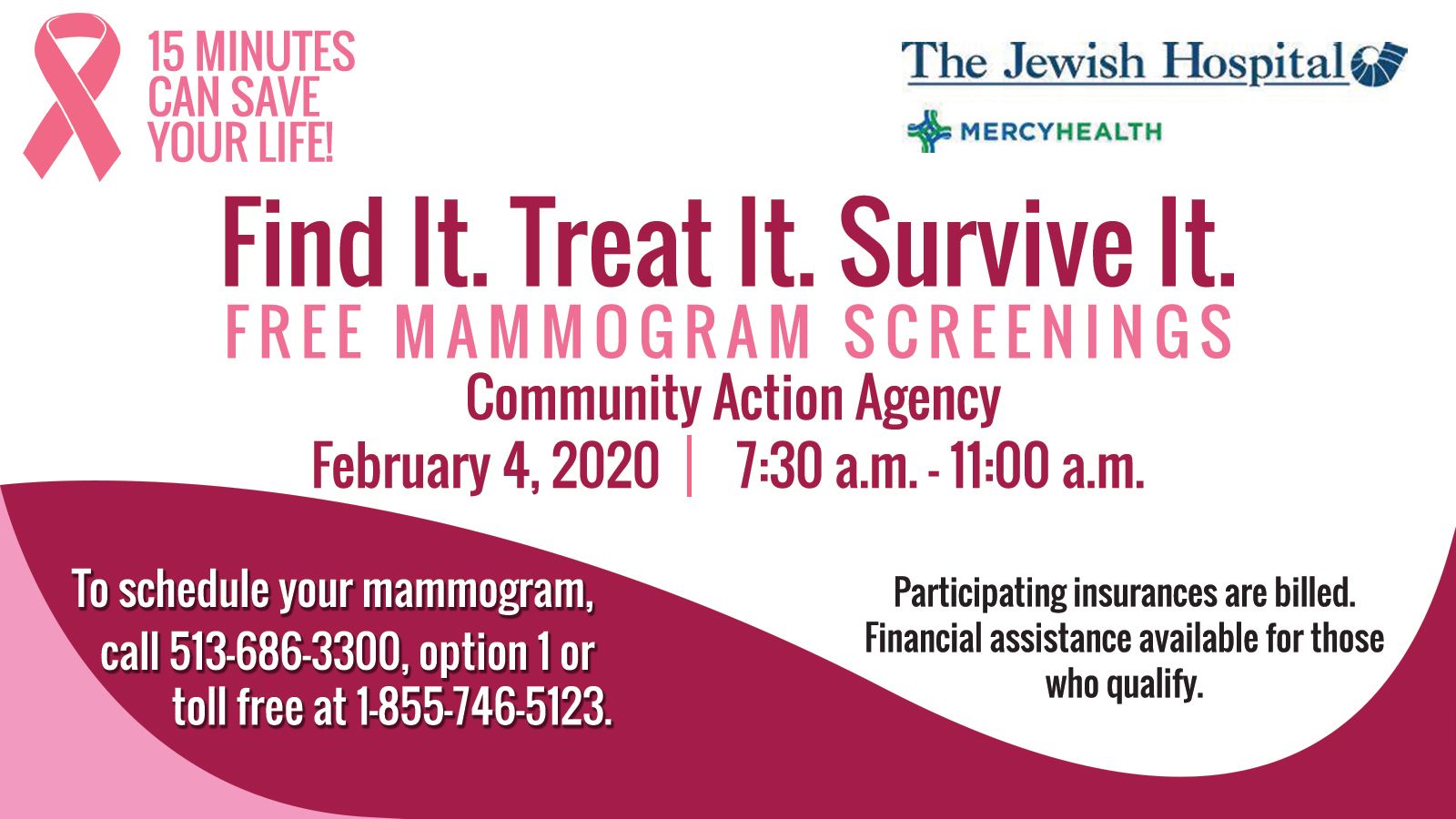This image is an informational business card-style advertisement with a primarily white background and accents of pink and red. Prominently, the top left corner features the pink ribbon breast cancer survivors logo with the slogan "15 minutes can save your life" in pink. In the upper right, it reads "The Jewish Hospital" accompanied by a shofar-like symbol, and below it, the cross logo of Mercy Health.

The central part of the card stands out with a bold message in red: "Find It, Treat It, Survive It." Below this, "Free Mammogram Screenings" is written in pink, followed by the details "Community Action Agency, February 4th, 2020, 7:30 a.m. to 11 a.m."

The bottom section of the card has a sweeping magenta or dark pink shape with a lighter pink wedge on the left. Text within this area provides contact information, reading: "To schedule your mammogram, call 513-686-3300 option 1 or toll-free at 1-855-746-5123." It also notes, "Participating insurances are billed. Financial assistance available for those who qualify."